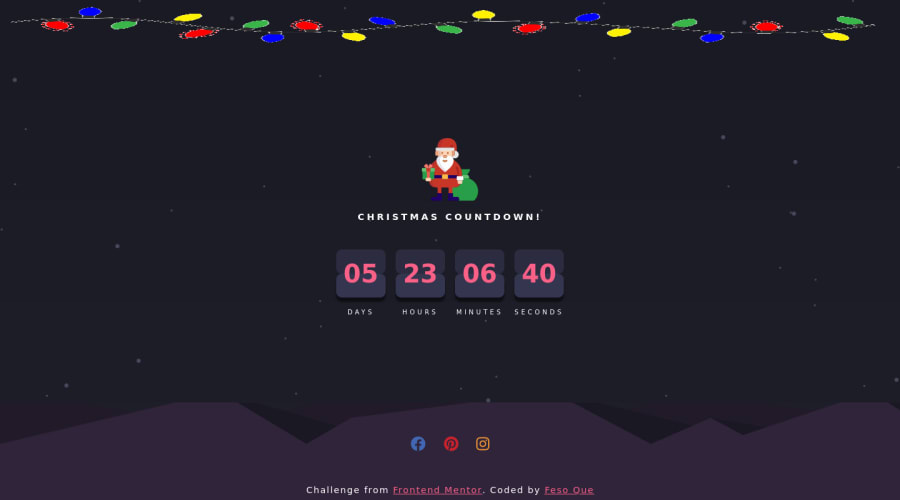The screenshot captures a visually appealing web page adorned with festive elements. The background is a deep, dark grayish-blue, setting a serene tone. At the top, a string of charming Christmas lights, featuring tiny oval-shaped bulbs in green, blue, yellow, and red, hangs horizontally. These bulbs are strung on a delicate gray line, reminiscent of holiday decorations typically seen on trees or houses.

In the center of the page, a small, detailed illustration of Santa Claus stands prominently. Santa is depicted holding a large green sack over his shoulder and a wrapped present in his hand, which is green with a red bow. Directly beneath this illustration, "CHRISTMAS COUNTDOWN" is written in small, white capital letters.

Below the title, a countdown timer is displayed in four distinct squares. The first square shows "05" in red, indicating the days remaining, with "Days" labeled beneath in small white letters. The second square features "23" in red for the hours left, labeled "Hours" below. The third square displays "06" for minutes, also with a "Minutes" label beneath. The final square counts down "40" seconds, labeled accordingly.

At the bottom of the image, a subtle depiction of a mountain range emerges in a lighter shade of gray, creating a contrast against the darker background. Centered above this range are three social media icons for Facebook, Pinterest, and Instagram.

Finally, the footer of the page includes text reading "Challenge from Front End Mentor," followed by "Coded by FESOQUE," indicating the creator of the page.